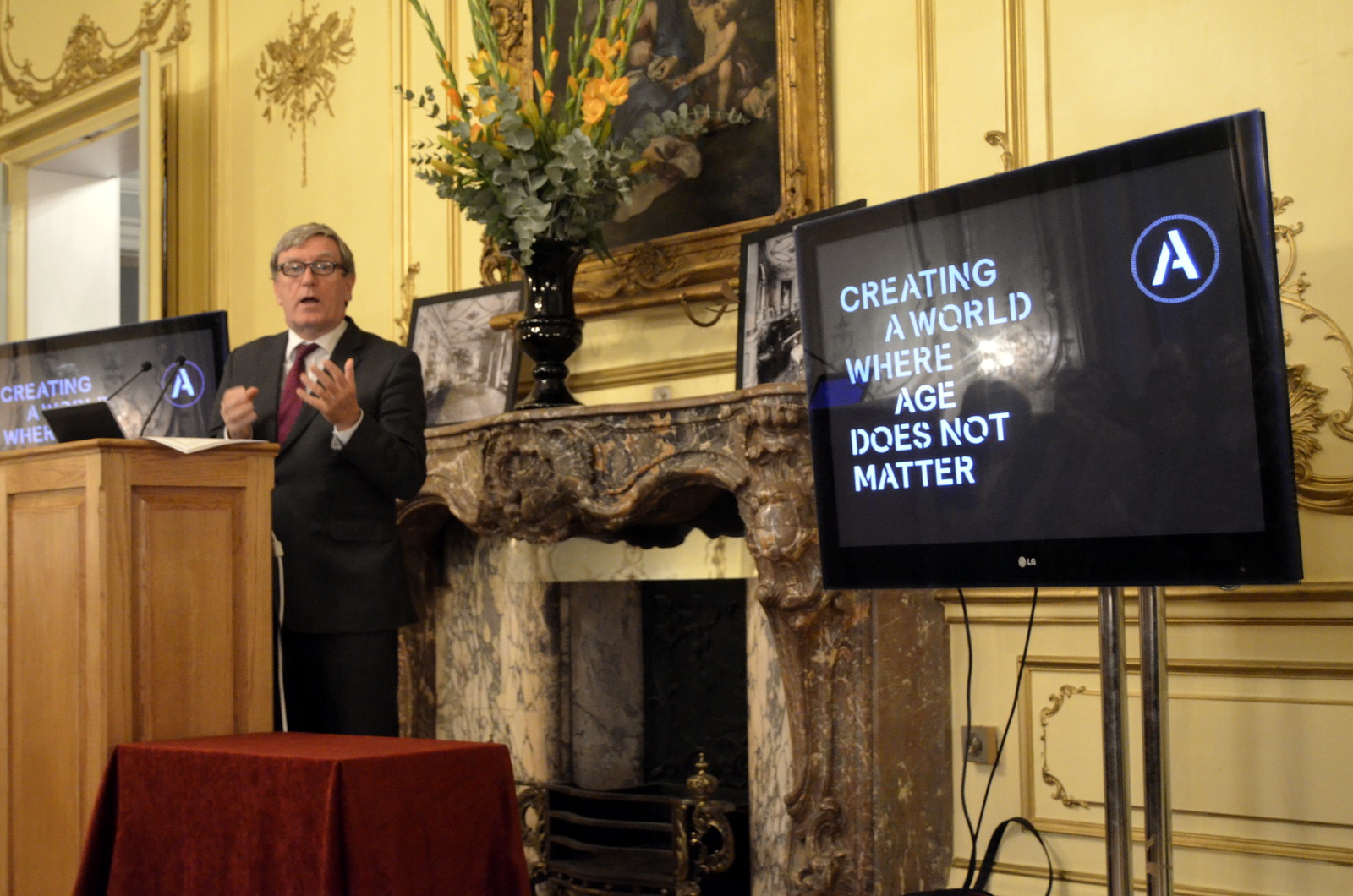The photograph, captured in a horizontal landscape orientation, features an older man presenting from a light brown wooden lectern on the left side of the image. He is dressed in a black suit, a dark red tie, and a white button-down shirt. With short gray hair and small glasses, he engages the viewer directly by looking into the camera while raising his left hand, likely emphasizing a point during his speech. Several microphones extend toward him from the lectern, where a laptop and papers are also visible.

Flanking him on either side are two flat-screen monitors with dark black borders, possibly LG-brand, displaying the text, "Creating a world where age does not matter," accompanied by a blue circle with a large white capital 'A' in the top right corner of the screens. 

The setting behind the man exudes opulence, with a prominent stone fireplace as the central feature, flanked by picture frames and a large vase filled with yellow flowers and green leaves. Above the fireplace hangs an ornate, old-fashioned gold picture frame, though the artwork inside it is indiscernible. The walls are painted yellow and adorned with gold molding, enhancing the posh, mansion-like ambiance of the room.